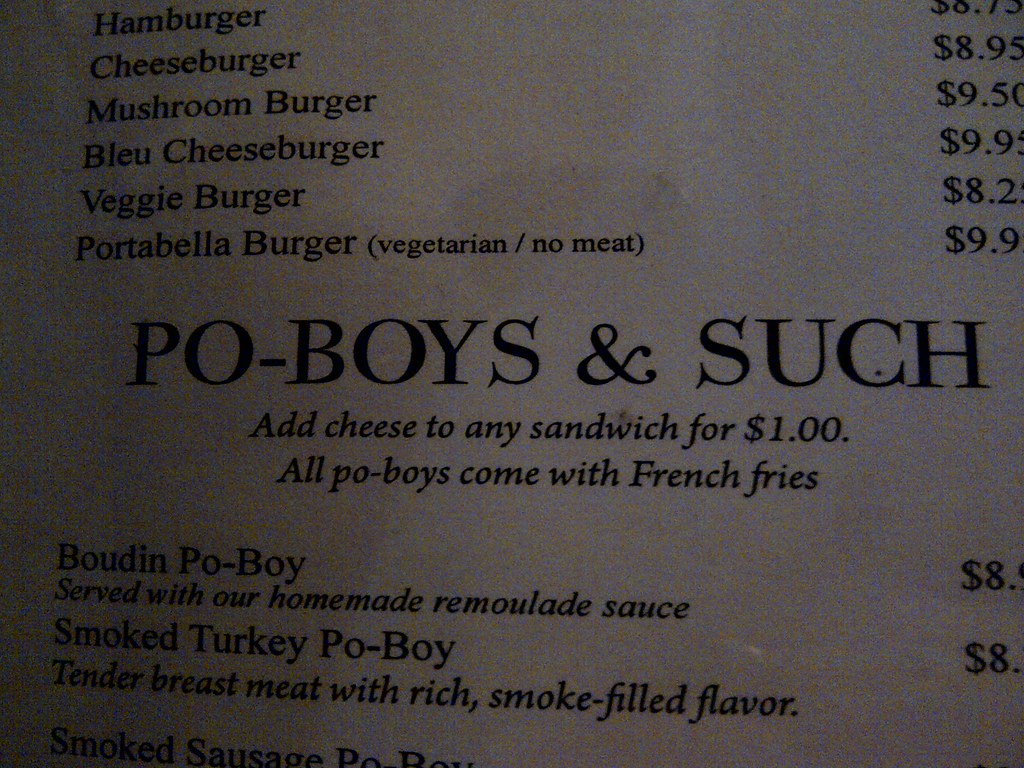This image features a partial menu set against a white background with black text. The menu lists various burgers with their titles and prices, although the price of the initial hamburger is cut off. The visible items and prices are as follows:

- Cheeseburger: $8.95
- Mushroom Burger: $9.50
- Blue Cheeseburger: $9.95
- Veggie Burger: $8.20
- Portobello Burger (vegetarian, no meat): $9.90

The menu also mentions an option to add cheese to any sandwich for an additional $1.

Following the burger section, the menu introduces "Po'boys and Such." All po'boys are served with French fries. Listed po'boys include:

- Pudding Po'boy served with homemade sauce: $8.00
- Smoked Turkey Po'boy featuring tender breast meat with a rich smoked filler: $8.00

The text indicates additional items regarding smoked sausage and other items, but the rest of the menu content is cut off in the image. This is a detailed glimpse into a diverse menu offering both classic and unique sandwich options.